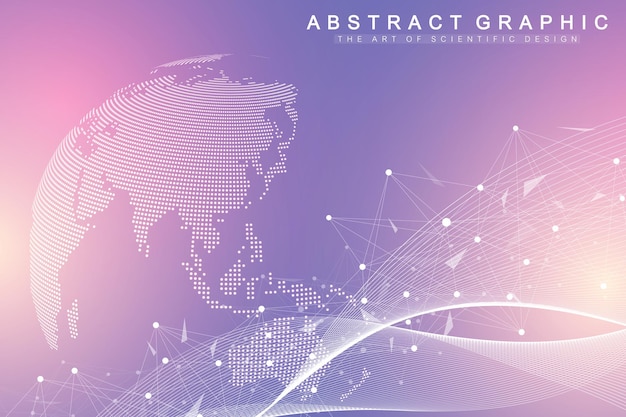The image is a professionally designed digital advertisement featuring a neon color scheme that transitions between pink, light blue, and purple shades. On the left side, there's an outline of a globe created with numerous small white dots. Towards the right, the design evolves into white curving lines and waves, interspersed with clusters of dots and triangles, resembling a network mind map. At the top right corner, the phrase "Abstract Graphic" appears prominently in white text, with "The art of scientific design" written below it, subtly highlighted in light gray. The entire composition showcases a blend of scientific and artistic elements, emphasized by sleek, thin typography and dynamic, interconnected patterns.